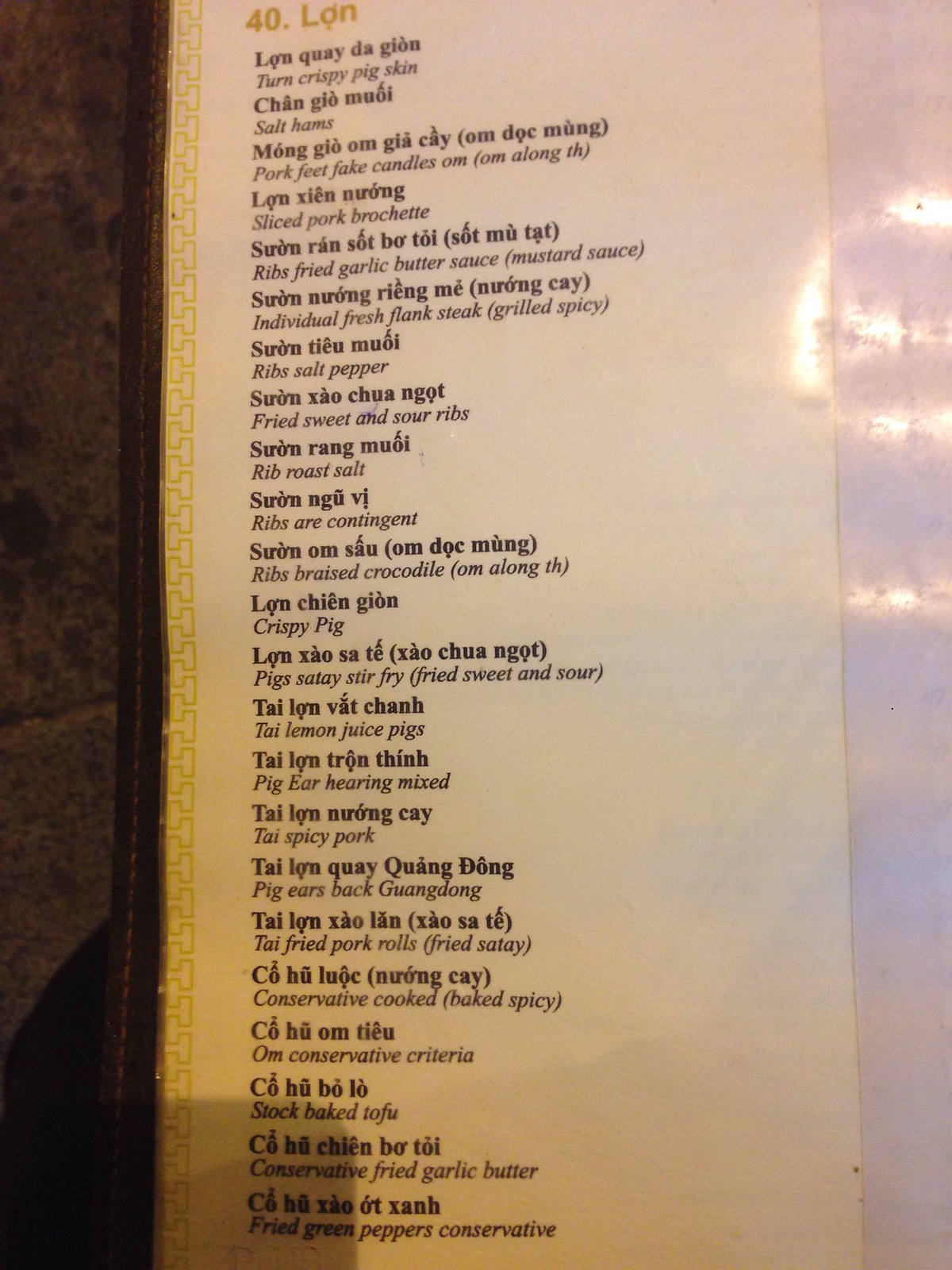The image displays a restaurant menu, meticulously laminated on a white paper with elegant leather-like trim around its edges. The menu is bilingual, featuring food items in both English and another language. Starting from the top, the English section lists various dishes such as Torn Crispy Pig Skin, Salt Hams, Pork Feet, Fake Candles, Sliced Pork Brochette, Ribs with Fried Garlic Butter Sauce, Ribs with Mustard Sauce, Individual Fresh Flank Steak Grilled Spicy, Ribs with Salt and Pepper, Fried Sweet and Sour Ribs, Rib Roast with Salt, Contingent Ribs, Ribs Braised with Crocodile, Crispy Pig, and Pig Satay Stir-fry, among others. Each delicious-sounding item promises a unique culinary experience, highlighting the restaurant's diverse and intriguing offerings.